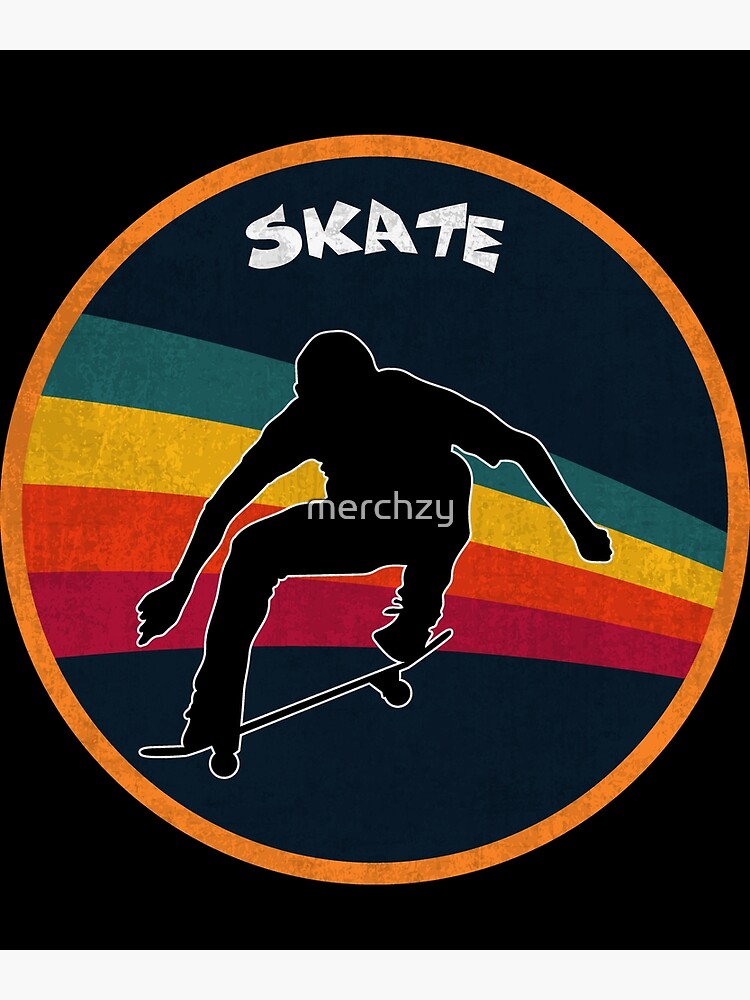The image features a skateboard-themed logo with a plain black background and a prominent orange circle in the center. Inside the orange circle, the word "SKATE" is written in bold, white uppercase letters at the top. A colorful rainbow, composed of dark green, yellow, orange, and a dark red or maroon, arcs across the middle of the circle, widening slightly as it extends from right to left. In front of this rainbow stands a hand-drawn silhouette of a skateboarder captured mid-jump, illustrated in black and outlined in white for contrast. At the top of the image, spanning across the skater, is the watermark "MERCHZY" written in lowercase letters, indicating it might be a brand or product related to skateboarding.